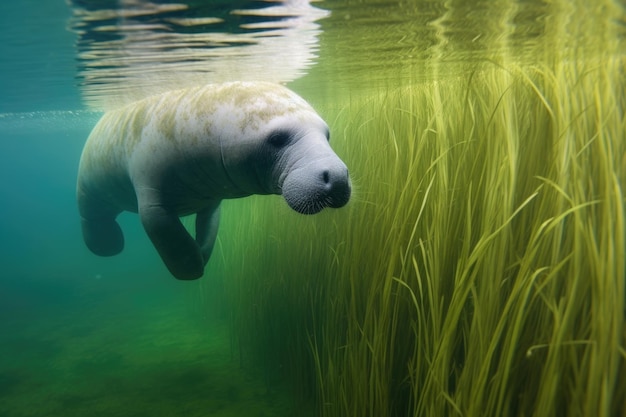An underwater scene features a manatee swimming close to the water's surface. The water is a striking mosaic of blue shades, from a deep turquoise transitioning to a blue-green towards the bottom. On the right side of the image, lush, bright green grass or weeds stretch upwards, some bending and waving gracefully under the water's current. These plants resemble a field of elongated, flowing wheat, adding to the scene's tranquil beauty.

The manatee, swimming from the left center towards the right, has a light gray, round body adorned with patches of green moss, particularly along its back and sides. Its distinct facial features include a wide, bulbous snout, whiskers, sunken eyes, and pronounced cheeks. The creature's flippers and tail are broad and paddle-like, helping it navigate the shallow, sandy waters. You can even see the manatee's reflection on the water's surface, adding depth and a sense of closeness to the serene underwater tableau.